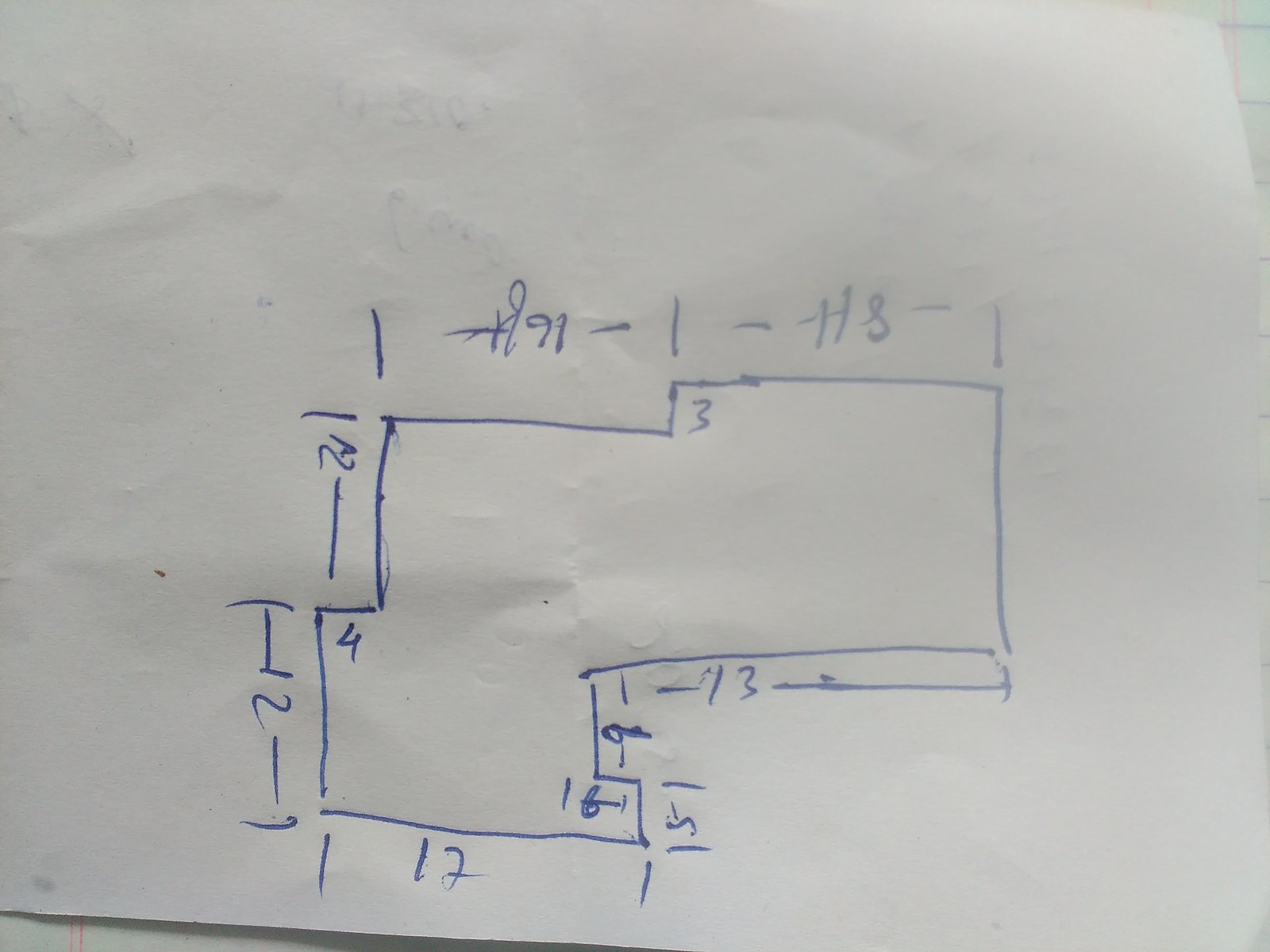The image features a hand-drawn sketch on white paper, rendered in blue ink. The drawing appears to depict an irregular, upside-down L shape, characterized by several sharp corners and non-linear edges. Along the outer lines, various numerical annotations are present, arranged with brackets and dashes for delineation.

Starting from the left side of the drawing:
- The outer line begins with the notation [−2] followed by −2 and 1.
- A dash precedes another number accompanied by a bracket, specifically [−2, 1].
- Continuing rightward, a sequence follows: −, 2, 1.

At the top width of the L shape:
- The sequence starts with a line, followed by a dash and the numbers 9 and 1.
- Subsequent numbers include: −1, −(88), and another dash leading to a downward-facing line.

On the right side and moving towards the bottom:
- At the bottom line, the sequence includes 13− followed by either −6 or −9 (depending on the orientation).
- This is followed by −15 and the number 12 at the end.

Within the shape, centrally located numbers include:
- 4 near the top-center,
- 3 in the middle,
- And 16 at the bottom.

This intricate diagram is meticulously annotated, possibly serving a specific technical or mathematical function, as indicated by the precise placement and variety of numerical values.